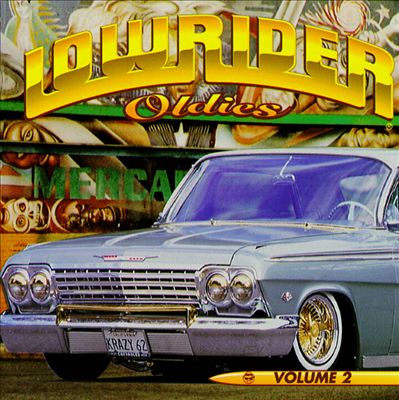The image appears to be an intricate and vibrant album cover for "Lowrider Oldies, Volume 2." Dominating the scene is a vintage blue Cadillac with an old-school design, flaunting gold-spoked rims and white-wall tires. The car's license plate reads "Crazy 62." The vehicle's imposing front grille is silver with an attached golden hue-piece, which stands out against the chrome silver bumper. Enveloping the top center of the image, gold letters with a gradient hue—from pure gold at the top to a lighter yellowish gold at the bottom—arrange to form the title "Lowrider Oldies," with the 'R' elegantly extending to the other letters.

The backdrop bustles with urban flair, featuring captivating graffiti reminiscent of Mexican and African art, including Mayan-like figures and the word "Mexicana." This art provides a rich, textured background for the featured car. At the bottom right, the album title "Volume 2" is inscribed, adding a final touch to the visually dense and culturally rich representation. Despite minor disruptions, like a pencil-shaped object under the right tire, the overall imagery remains compelling and evocative, suggestive of the vibrant, retro essence of Lowrider culture.